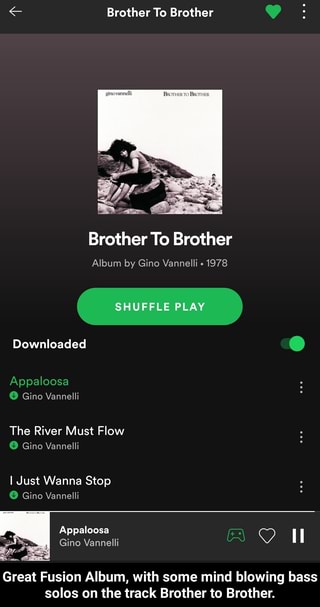The image depicts a Spotify album interface showcasing the album "Brother to Brother" by Gino Vannelli. At the top of the interface, there is a dark gray strip with bold white text reading "Brother to Brother," with "B" and "T" capitalized. On the left side of the strip, there's a left-pointing arrow, and on the right, a green filled heart indicating that the user has liked the album. Further to the right, three white dots signify a submenu option.

The background starts as a lighter grayish-purple at the top and gradually fades to black towards the bottom. Centered on the page is the album cover, which features a grayscale image of what appears to be a woman picking up rocks at the beach, set against a white background. Below the album cover, the artist's name "Brother to Brother" is prominently displayed in bold white text, with a smaller, light gray text underneath indicating "Album by Gino Vannelli" and a bullet point followed by "1978."

Below this section, there is a conspicuous green oval button that reads "SHUFFLE PLAY" in white capital letters. To the left of this button, the word "Downloaded" is visible, and to the right, a toggle switch is turned on, indicated by a green circle. Beneath this section, green text reads "APPALOOSA" with the artist's name in gray underneath. To the left, a green circle containing a downward-pointing arrow indicates a download symbol. To the right of this, three circles hint at additional options.